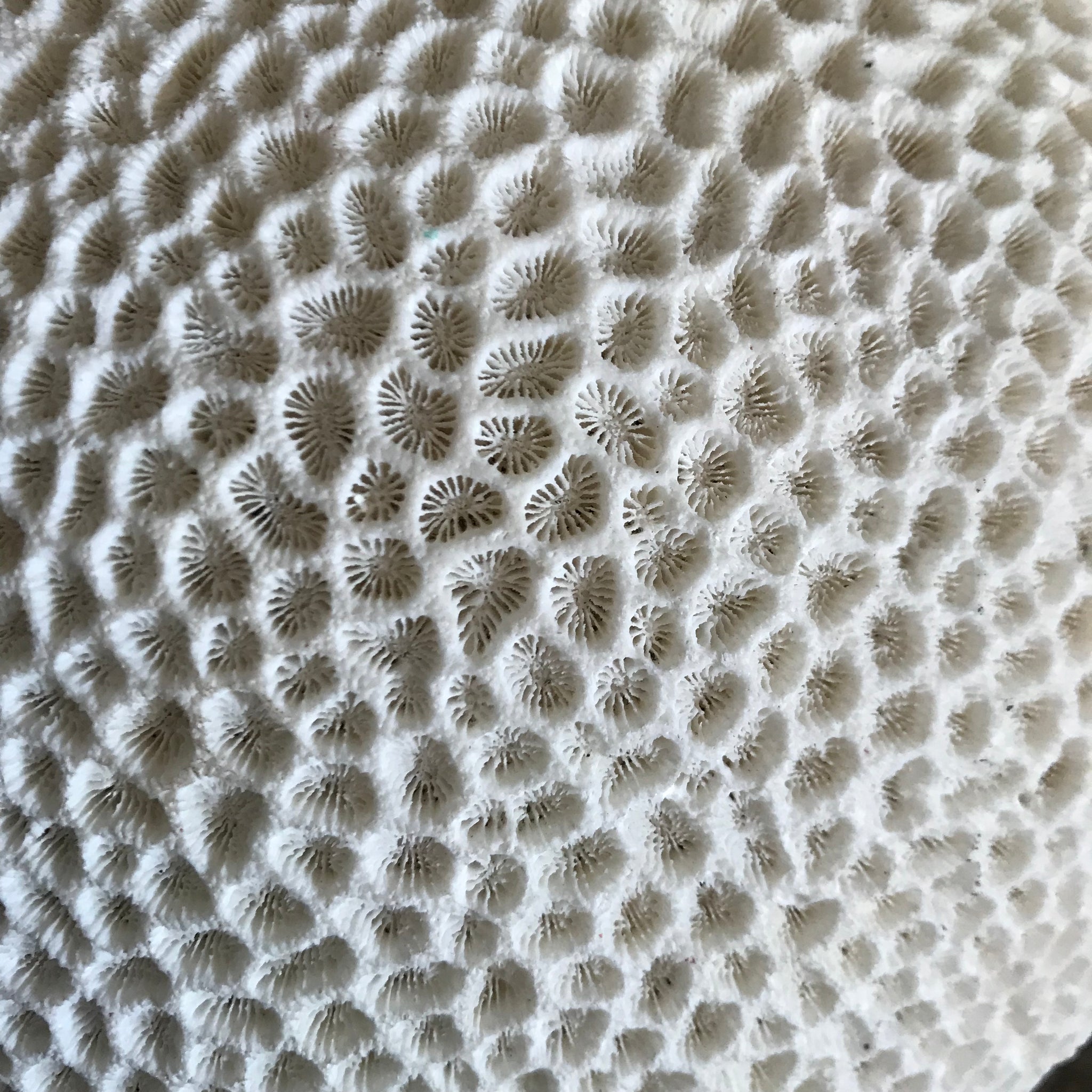The photo depicts a highly detailed, close-up view of a porous, fossilized surface resembling a section of desert ground. The entire image is dominated by a white to cream-colored texture, riddled with numerous irregularly shaped holes scattered across the surface. Inside each hole, intricate, tiny squiggly black lines extend from the borders toward the centers, creating a complex, web-like pattern within each indentation. These lines are reminiscent of fossilized sea creatures, possibly sea urchins. The texture of the surface appears to have a relief effect, where the recessed areas seem darker, almost like nodes pulling the surface inward. The perspective is nuanced, making it difficult to discern whether the features are protruding or hollowed out. At the bottom of the photo, there's a black corner, suggesting a possible cross-section of the ground. This fascinating, science-book-esque image captures the multi-faceted, textured nature of the fossils against the contrasting creamy background.